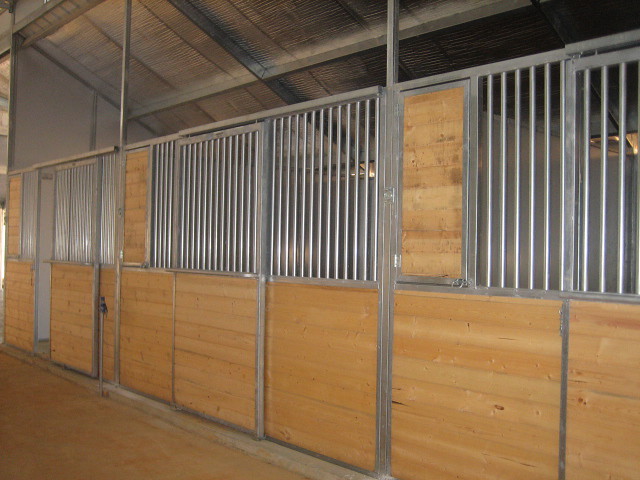This is a photograph of the interior of a high-quality, professional horse barn, taken from the center aisle. The stable features a veed, slanted roof likely made from corrugated steel, and the aisle floor appears to be a clean, brown dirt or sand. The stables, crafted from light-colored wood on the lower half, are panelled with vertical silver bars on the upper half to ensure the horses' safety and prevent them from jumping out. Each stable has a sliding door, with one in the distance shown open, revealing a white wall and no horses in sight. The aisles and stables are meticulously clean, conveying the overall sophistication and expense of this well-maintained horse barn.